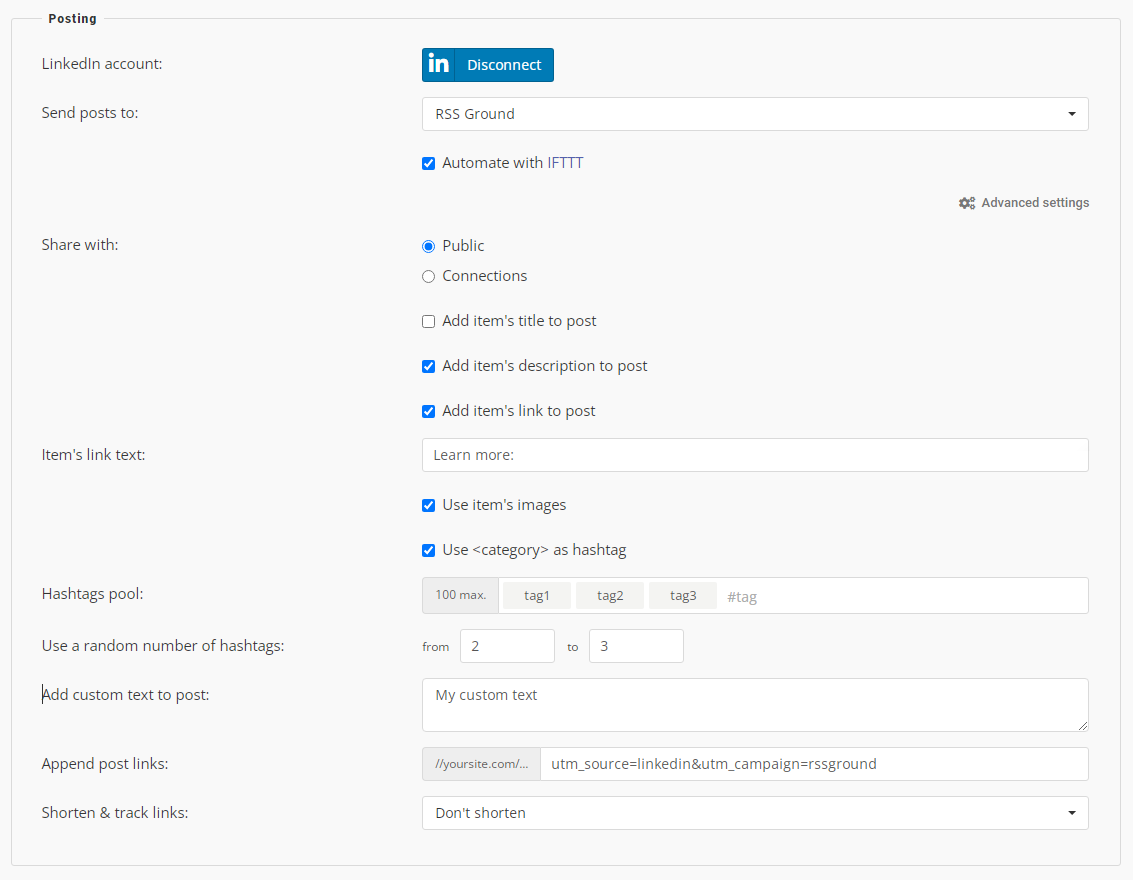The image displays a slightly wider-than-tall settings interface, likely from LinkedIn, against a light gray background. At the top, there is a heading titled "Settings." 

On the left-hand side, the section begins with "LinkedIn Account:" followed by the LinkedIn logo—a blue square with "IN" in white. Adjacent to this logo is a blue button labeled "Disconnect," suggesting the option to disconnect the LinkedIn account.

Below this, a section labeled "Send post to:" features a drop-down menu with "RSS ground" selected. Directly beneath, a checkbox labeled "Automate with IFTTT" is marked with a blue check. 

Further down the interface, on the right-hand side, there is a gear icon labeled "Advanced Settings." 

Additionally, another section labeled "Share with:" offers two selectable bubbles. The "Public" option is currently selected, while the alternative "Connections" option appears below.